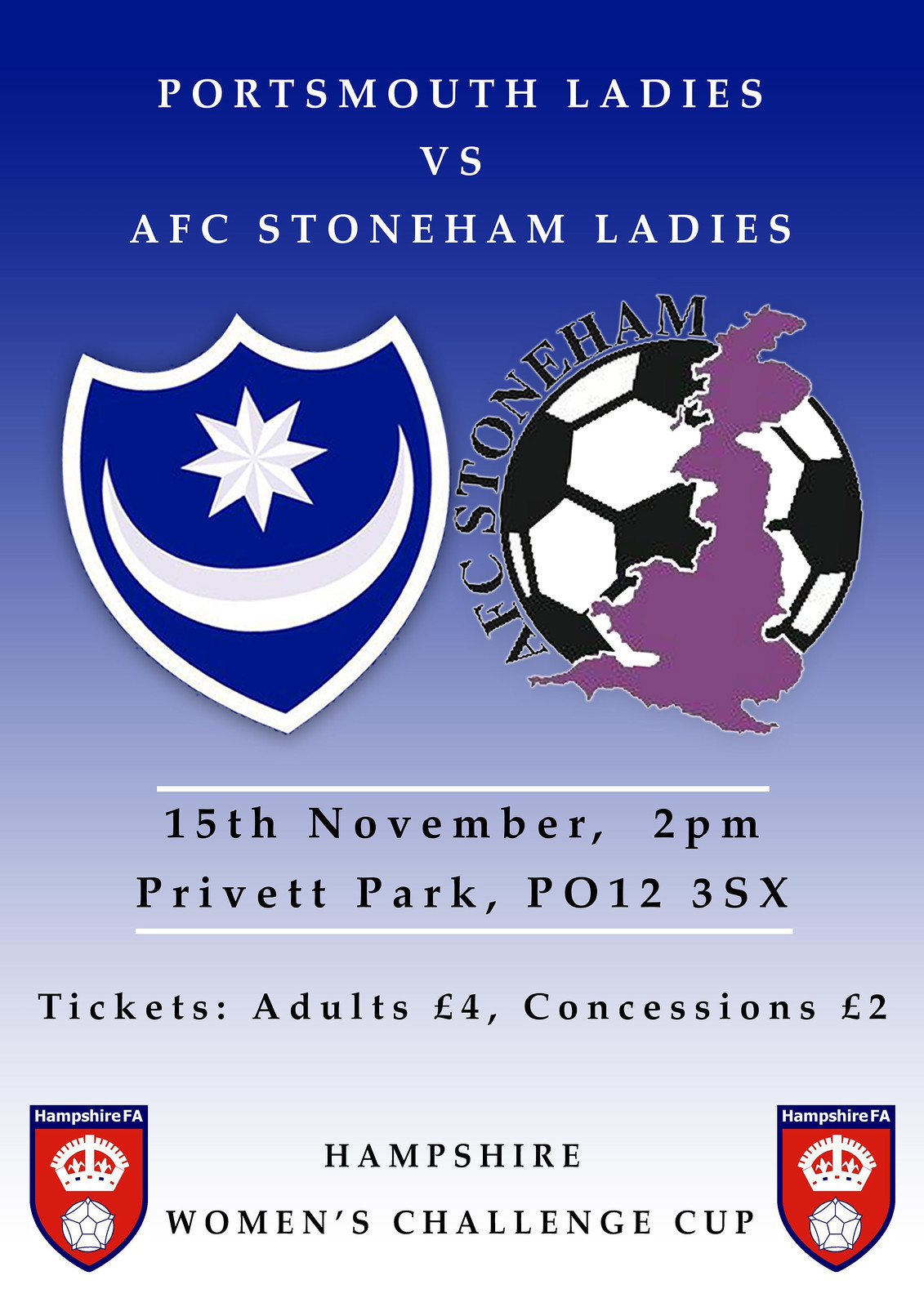This is a visually striking poster promoting a soccer match between Portsmouth Ladies and AFC Stonem Ladies. The poster features a gradient background that transitions from royal blue at the top to a lighter blue in the middle, eventually fading to white at the bottom. At the top of the poster, "PORTSMOUTH LADIES VERSUS AFC STONEM LADIES" is prominently displayed in bold, white, all-caps text.

Below the title, on the left side, is a detailed crest with a royal blue shield accented by white trim. The shield features a white crescent moon at the bottom, with its tips pointing upward, and an eight-pointed white and gray star above the moon. To the right of the crest, there is a soccer ball with black and white patches. Imprinted on the ball is a purple silhouette of England, and encircling the ball in black text are the words "AFC STONEM."

Further down the poster, key event details are provided in black text: "15th November, 2 P.M., Privet Park, P.O. 123SX." Information on ticket prices follows, stating "Tickets: Adults £4, Concessions £2." The poster concludes with the announcement of the "Hampshire Women's Challenge Cup," flanked on either side by two Hampshire logos. Each Hampshire logo features blue, red, and white colors, and includes a crown as well as a circle containing a star.

Overall, the poster effectively conveys all necessary information with clear typography and distinct team graphics.